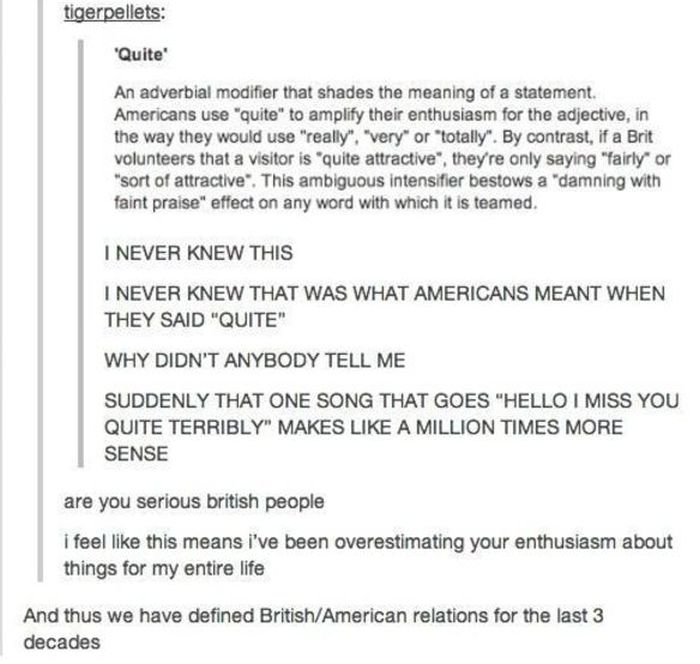This screenshot from a forum page features a discussion revolving around the differing usage and interpretation of the word "quite" between Americans and Brits. The background of the page is white, and all text is in black font. 

At the top, the username "Tiger Pellets" is followed by a colon, introducing their response.
The response begins with a bolded title "Quite", followed by a detailed explanation in regular black font. It reads: 

"An adverbial modifier that shades the meaning of a statement. Americans use 'quite' to amplify their enthusiasm for the adjective in the way they would use 'really,' 'very,' or 'totally.' By contrast, if a Brit volunteers that a visitor is quite attractive, they're only saying fairly or sort of attractive. This ambiguous intensifier bestows a 'damning with faint praise' effect on any word with which it is teamed."

Following this explanation, "Tiger Pellets" continues with a personal reaction:

"I never knew this. I never knew that was what Americans meant when they said 'quite.' Why didn't anybody tell me? Suddenly that one song that goes, 'Hello, I miss you quite terribly,' makes like a million times more sense."

Below this, another comment from "Tiger Pellets" is separated by a vertical gray line. This comment continues:

"Are you serious, British people? I feel like this means I've been overestimating your enthusiasm about things for my entire life. And thus we have defined British-American relations for the last three decades."

The visual layout suggests that the forum is structured with nested comments and replies, illustrated by the vertical gray lines connecting "Tiger Pellets" to other user interactions.